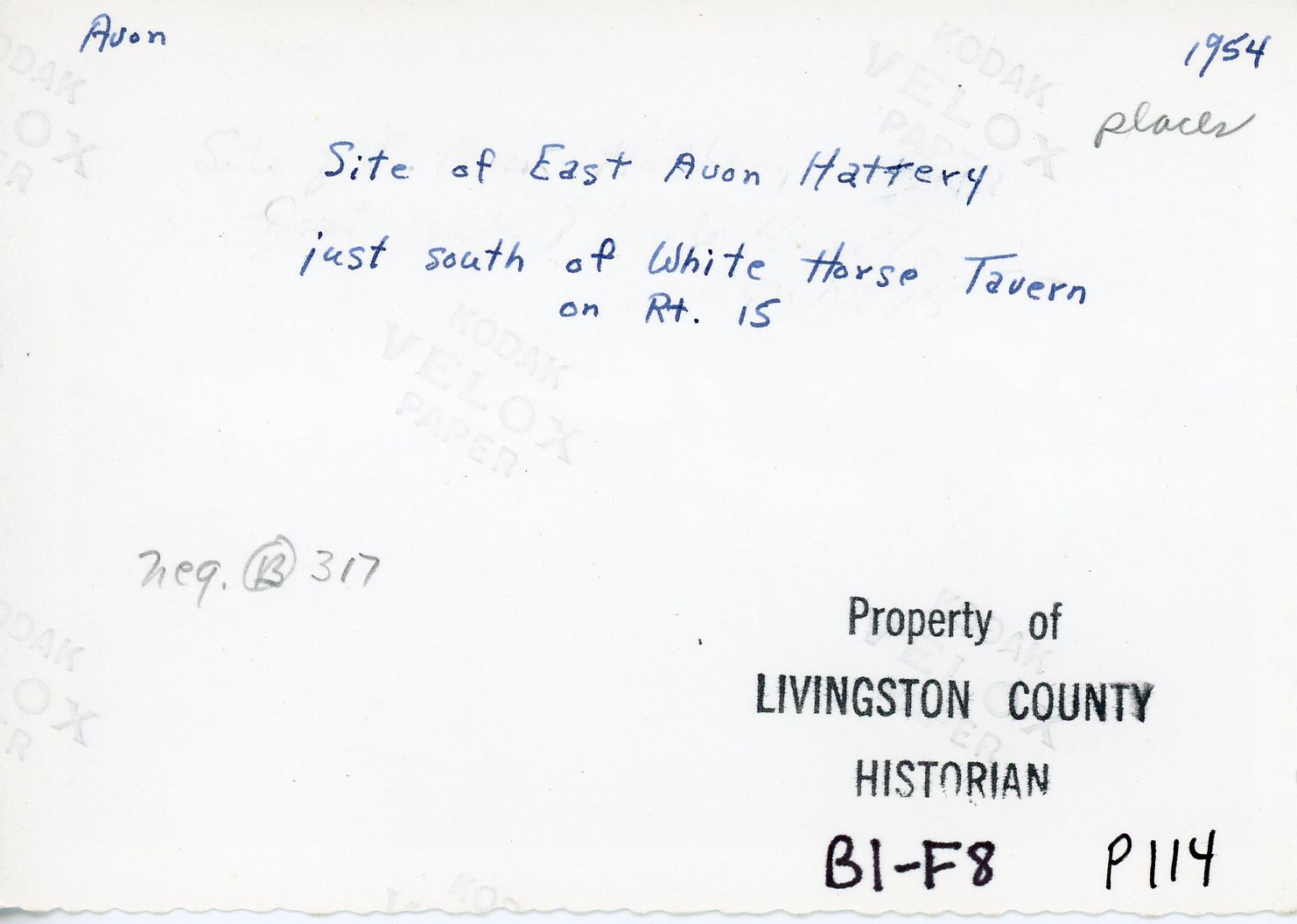The image is a scan of a white piece of paper, likely the back of a photograph, given the repeating watermark that says "Kodak Velox Paper." This suggests the paper is from Kodak, a well-known camera company. In the upper middle of the paper, there is light blue handwritten text that reads, "Site of East Avon Hattery just south of White Horse Tavern on RT 15," dated 1954. The upper right corner also contains blue pen text with the same year, "1954." To the upper left, more blue pen handwriting simply states, "Avon." In the bottom middle left, there is light pencil writing that says, "neg B 317," with the letter "B" circled. The lower right corner features a black stamp that reads, "Property of Livingston County Historian." Below the stamp, there is heavy black pen or marker text with the notation, "B 1-F 8," and to the right of that, "P 114." The handwritten notes appear to be in various styles and formats, adding to the historic and archival nature of the document.